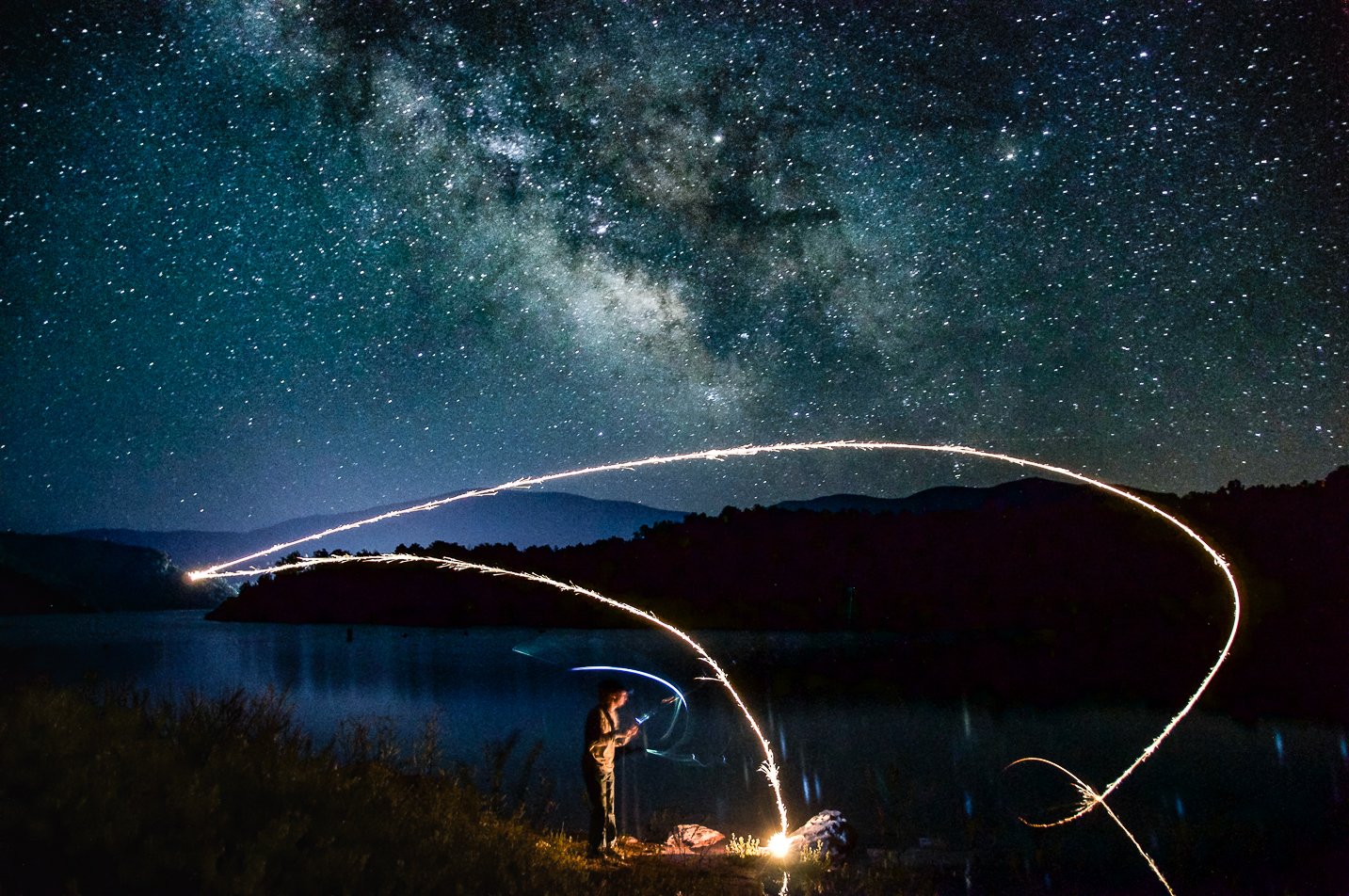In this hyper-realistic and digitally manipulated night scene, a man stands at the shoreline of a serene body of water, foregrounded by a mountain range silhouetted against the dark horizon. He is positioned next to a small campfire, which casts a warm glow around him. The night sky above is beautifully detailed, featuring the vibrant, star-studded expanse of the Milky Way, interspersed with intricate blue, green, and white nebula patterns. The man appears to be engaged in a creative light display, spinning a ball of steel wool that's been ignited. Captured through a long exposure time-lapse, the luminous paths created by the burning steel wool swirl and arc majestically across the sky, reminiscent of sparkler trails. The dark, almost black sky enhances the stunning light effects and the celestial backdrop, making it a captivating blend of nature, fire, and artistic light play.